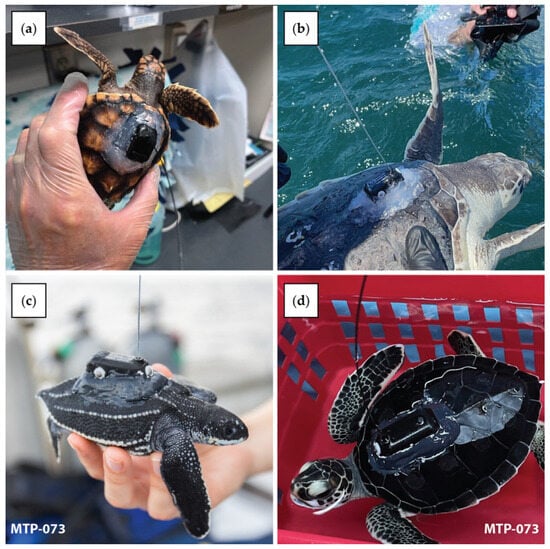The image comprises four distinct scenes, labeled A, B, C, and D, each showcasing a different sea turtle. Scene A features a small turtle with a brown and black patterned shell, marked notably in the center with what appears to be a black patch surrounded by silver, possibly a tracker or life support device. This turtle is being held in a person's left hand, which is white-skinned, possibly in a laboratory setting. Scene B shows a larger turtle being lifted from the water, exhibiting a gray and white coloration and a gray shell. In scene C, there is a smaller, black-shelled turtle with white dots along its back, held by someone's hand. Lastly, scene D presents another turtle with a black, shiny shell placed inside a red shopping basket.